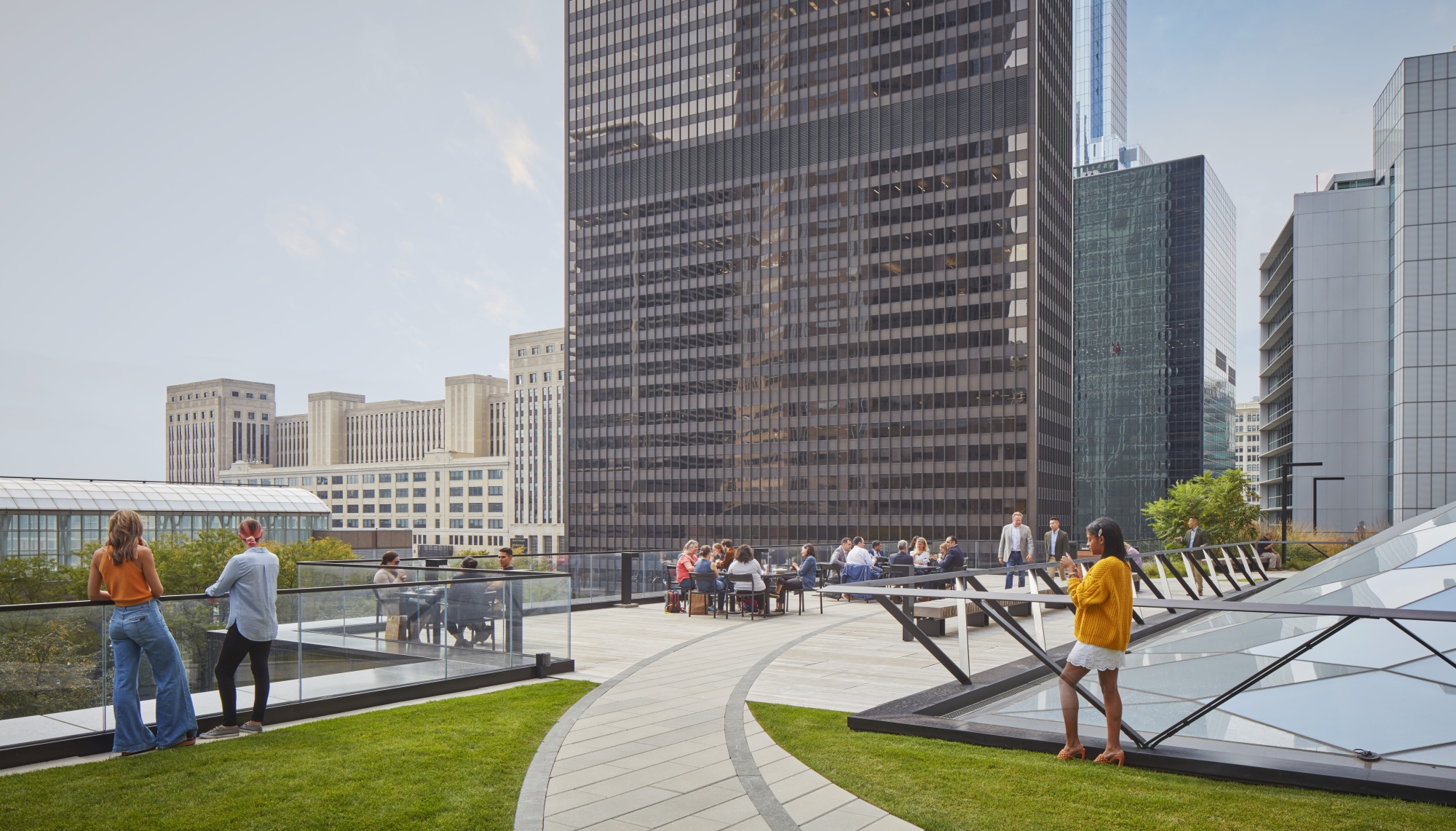This daytime photograph captures a bustling cityscape focused on a business district. Dominating the background are a series of tall buildings, predominantly with glass fronts, including an exceptionally large central building extending beyond the frame. In the foreground lies an open social gathering area, designed with a mix of paved pathways and manicured lawns. The stone pathway arches forward from the green grassy area at the bottom and leads to a larger, rectangular standing area, enclosed by waist-height glass barriers.

Scattered throughout are various seating arrangements: park benches, tables, and rectangular stone seating. Groups of people are seated at tables, with some tables holding up to ten individuals; others are standing or walking around, including one solitary woman and diverse groups of men and women of various backgrounds. The scene is vibrant with human activity against the backdrop of a hazy, yet bright sky.

To the left, two individuals gaze out towards the city, while to the right, a lone person stands near a raised, fancy glass feature. Distant greenery, including bushes and trees, and possibly a glass-encased arboretum or greenhouse with arching windows, add a touch of nature to the urban setting. This visually dynamic image contrasts the towering architecture with the communal, verdant foreground, capturing the essence of urban life during a bright, though not perfectly clear, day.